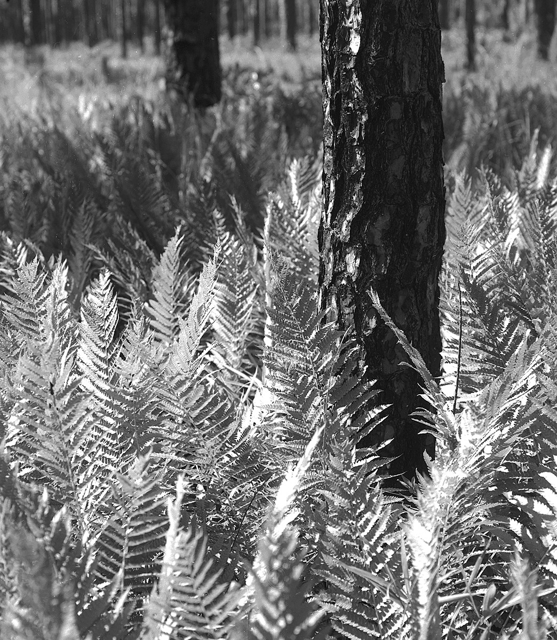This black-and-white outdoor photograph, taken in portrait orientation, offers a close-up view of a field brimming with tall ferns and rugged tree trunks. The scene captures a heavily wooded area where several pine trees, their tops cut off by the frame, rise from a forest floor blanketed with upright ferns. The foreground highlights one particularly detailed tree trunk to the right, its rough, textural bark starkly defined and partially glistening in the sunlight. The ferns surrounding it boast long, offshooting leaflets, stretching several feet tall and densely populating the scene. In the distance, additional tree trunks dot the landscape, reinforcing the sense of a vast, verdant forest floor. Overall, this photograph embodies a sense of realism, showing nature in its raw, unfiltered state.